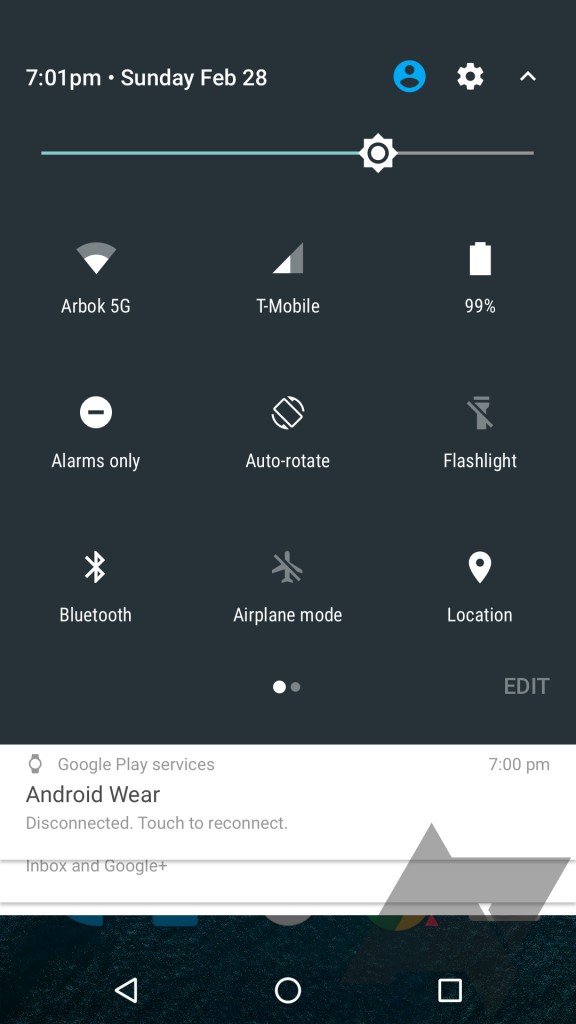A screenshot of a smartphone display shows a predominantly black background showcasing various icons and status indicators. At the very top, the current time is displayed as 7:01 p.m., alongside the date, Sunday, February 28th. To the right of the date and time, there is a blue bubble icon with a person symbol, a settings gear icon, and an upward arrow.

Below this top row, there is a horizontal slider featuring a settings gear icon, positioned approximately three-fourths to the right. Underneath the slider, "Arbok 5G" appears next to a Wi-Fi symbol, indicating network connectivity. To its right, "T-Mobile" is displayed accompanied by a triangle signal symbol, followed by a battery icon showing 99% charge.

Further down, under the Wi-Fi information, icons for various phone settings are displayed. "Alarms Only" is labeled along with a white circle containing a black dash, indicating that the phone is set to alarms-only mode. Adjacent to this is the "Auto-Rotate" setting with a rotating phone symbol, and "Flashlight" next to a flashlight icon.

The next row includes "Bluetooth" shown with its respective symbol, "Airplane Mode" with an airplane icon, and "Location" featuring a pin symbol. This layout suggests that it is one of two pages, allowing users to swipe right for more options.

At the bottom of the screen, a white banner notifies the user that "Google Play Services" was accessed at 7:00 p.m. Additionally, it states "Android Wear disconnected" with a prompt to "touch to reconnect."